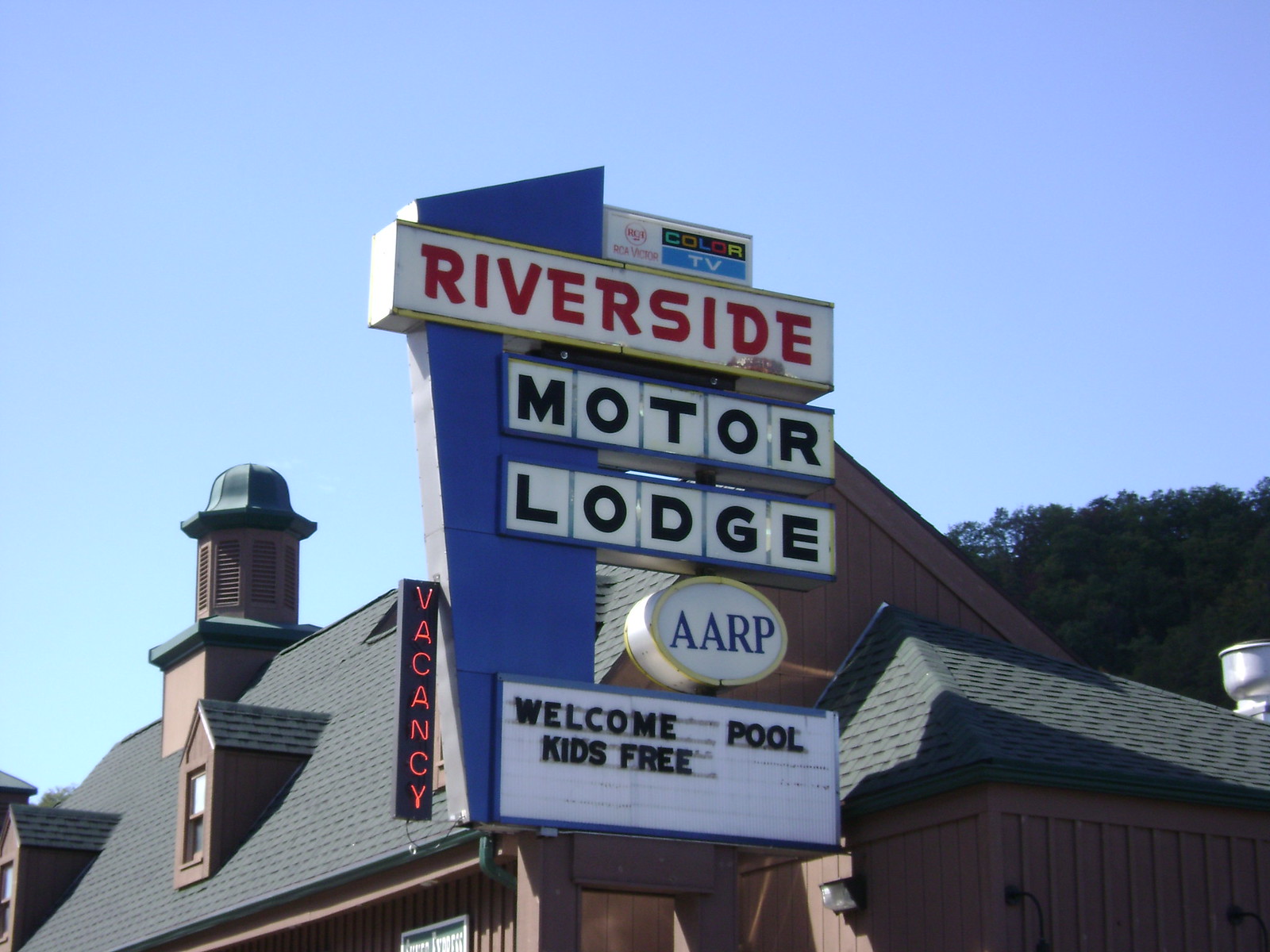The image showcases an old-fashioned motel sign for the "Riverside Motor Lodge." The sign is tilted slightly to the right and features several distinct sections. At the top, a white box contains a black box with the word "color." Below that, a blue box displays the letters "TV." Further down, a prominent white section is accentuated by yellow lines at the top and bottom, with the word "Riverside" in bold red text at its center. Underneath, two rows of five white squares each spell out "Motor" and "Lodge" in black letters.

An oval with a yellow rim follows, containing the blue letters "AARP." Beneath this, another white square with black text reads "Welcome Pool Kids Free." Attached to the left side of the main sign is a black rectangle with red illuminated letters that say "Vacancy."

In the background, the roof of the motel is visible, marked by dark gray shingles and a distinctive dome structure further to the left. On the right side, the backdrop includes very dark green trees against a clear blue sky.

The overall atmosphere is welcoming, with a distinct retro vibe reminiscent of the 1950s. The motel's walls and siding are painted black with green accents. The sky is bright and blue, indicating a pleasant day.